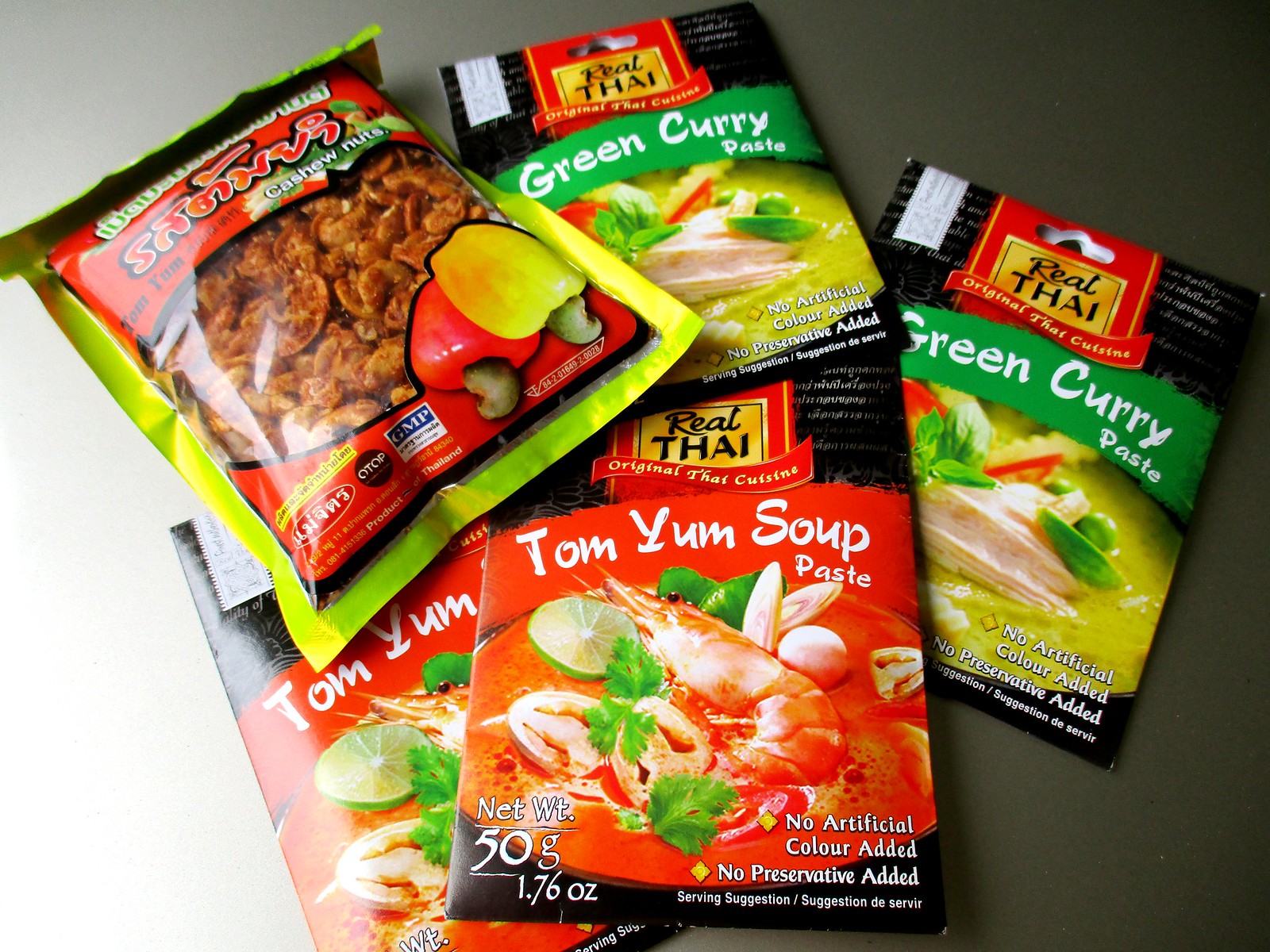The image displays an assortment of five Real Thai culinary products arranged on a smooth, dark surface that transitions from green on the right to white on the left. Dominated by a black color scheme, the packaging prominently features the company's logo, "Real Thai," along with the slogan "Original Thai Cuisine" on a red ribbon. Two packets of Tom Yum Soup Paste and two packets of Green Curry Paste, all black with their respective names in white text, are at the forefront. The Tom Yum Soup Paste packages showcase a vibrant image of soup containing prawns, lime slices, and various vegetables, emphasizing its authentic flavor. The Green Curry Paste packages depict a savory green curry dish with chicken. On the left, there is a packet of spiced cashew nuts in a green package with a red banner and a transparent window revealing the nuts inside. Each package clearly states "No artificial color added," "No preservative added," and "Serving suggestion," with the net weight displayed in white on the bottom left corner. Realistic images of bell peppers and other fresh ingredients enhance the appeal of these traditional Thai cooking essentials.